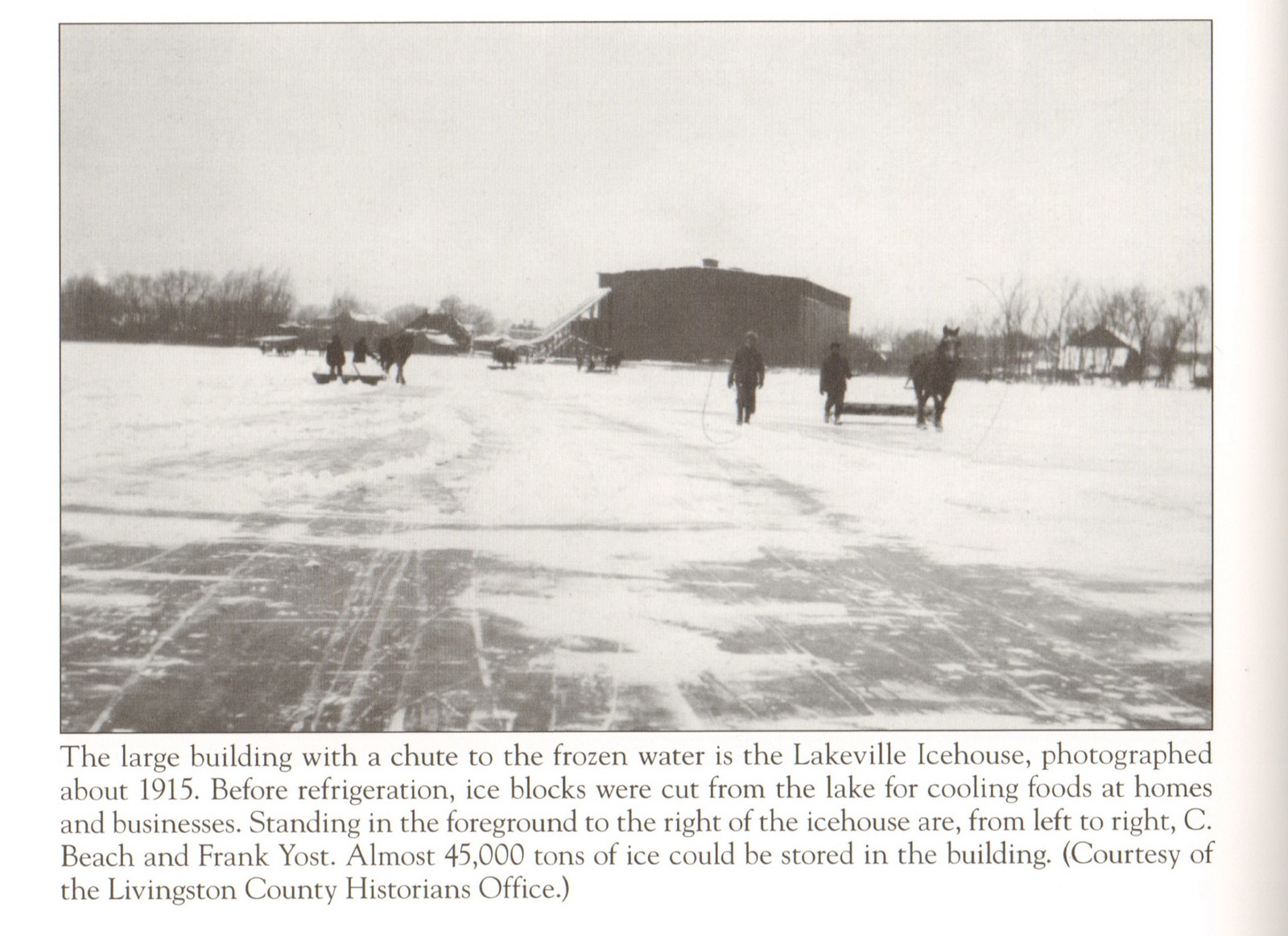This black and white photograph, taken around 1915 and printed in an older book, captures a snowy landscape where several individuals are seen walking across the frozen terrain. Prominently, the Lakeville Ice House stands in the background, recognizable by its chute leading to the frozen water. This large building, capable of storing almost 45,000 tons of ice, was essential for cutting ice blocks from the lake to cool foods in homes and businesses before the advent of refrigeration. The scene also includes a horse pulling a log of wood, and standing in the foreground to the right of the ice house are, from left to right, Sea Beach and Frank Yost. The tree line composed of very thin trees adds to the historical essence of the image, which is documented courtesy of the Livingston County Historian's Office.